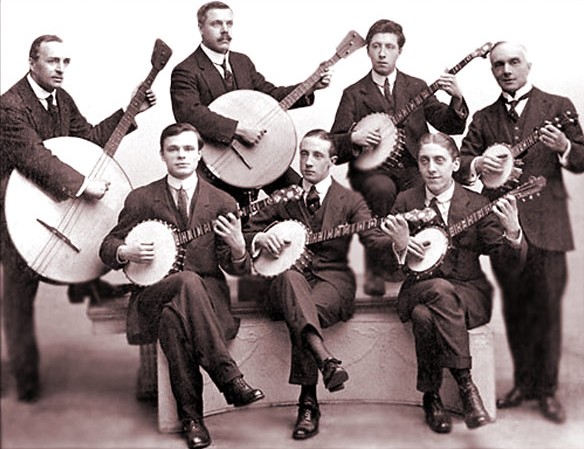The black and white photograph features a seven-piece banjo band, most likely from the late 19th or early 20th century. The ensemble consists of white gentlemen dressed in black suits, black dress shoes, white dress shirts, and black ties. They all have short, clean-cut hairstyles, with a few sporting facial hair, notably one man with a mustache in the top center of the image. The men are arranged with four standing in the back and three seated in the front on a bench, all holding banjos of varying sizes. The largest banjo is held by the gentleman on the far left in the back row, with progressively smaller banjos held by each subsequent person. The three men in the front are sitting with their legs crossed, each handling medium-sized banjos. The combination of their attire, the instruments, and the photo style suggests a formal, early 20th century European or American musical group.